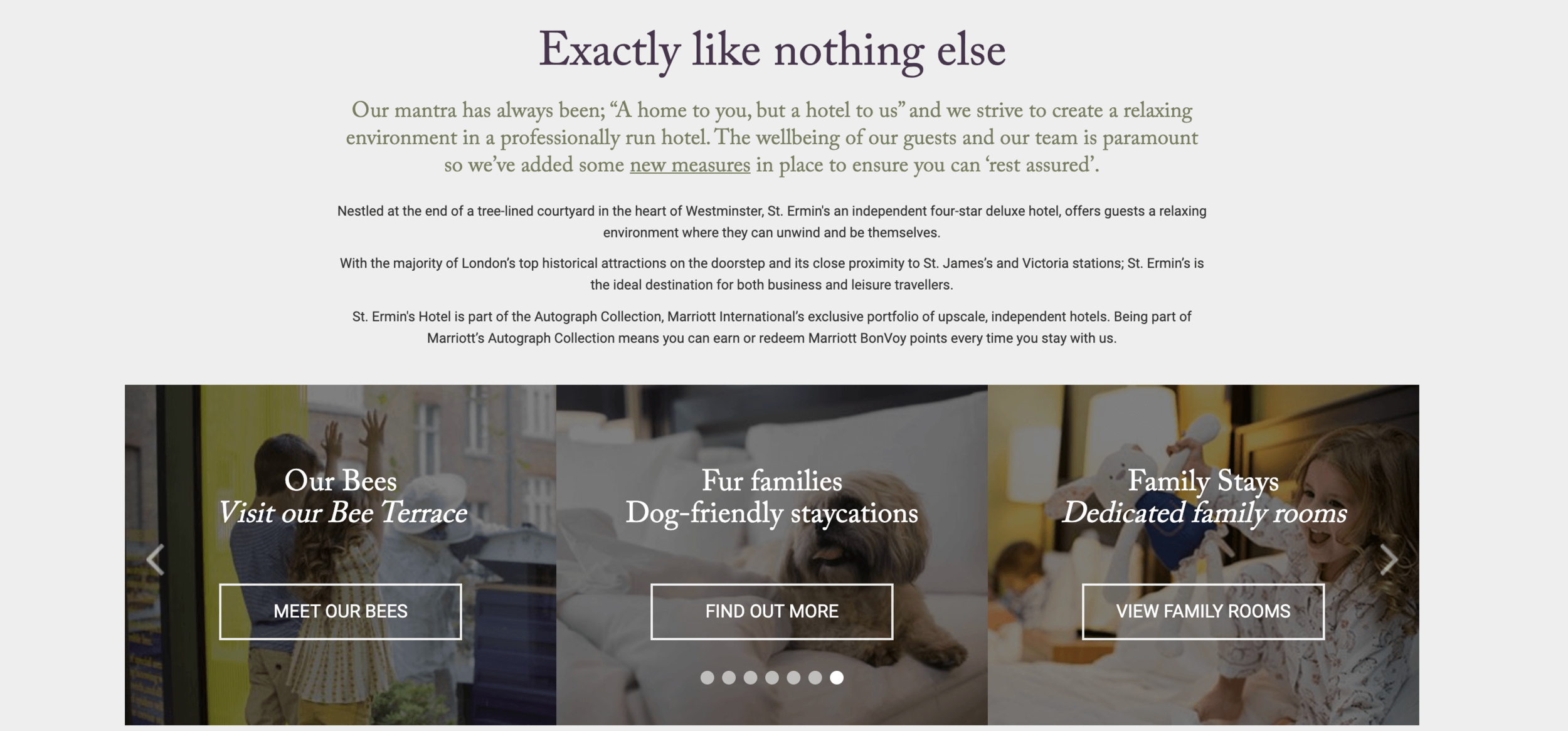This landscape-oriented advertisement appears to be sourced from a webpage, predominantly featuring a gray background. The layout is approximately twice as wide as it is tall, with various elements strategically placed to convey a comprehensive message.

At the top center, in bold black font, the text reads: "Exactly Like Nothing Else." Below this, in smaller green font, it states: "Our mantra has always been 'a home to you, but a hotel to us.' We strive to create a relaxing environment in a professionally run hotel. The well-being of our guests and our team is paramount, so we've added some new measures to ensure you can rest assured."

Notably, "new measures" is underlined for emphasis.

In the smallest black font, nestled towards the end of the advertisement, it reads: "Nestled at the end of a tree-lined courtyard in the heart of Warminster Street, your amenities are well provided. This independent four-star deluxe hotel offers a relaxing environment where guests can unwind and be themselves. With the majority of London's top historical attractions on its doorstep and close proximity to St. James and Victoria Station, St. Hermann's is the ideal destination for both business and leisure travelers."

Continuing, it further articulates: "St. Hermann's Hotel is part of the Autograph Collection, Marriott International's exclusive portfolio of upscale independent hotels. Being part of Marriott's Autograph Collection means you can earn or redeem Marriott Bonvoy points every time you stay with us."

At the bottom of the advertisement, there are three images depicting people, dogs, and other scenes, likely highlighting the hotel's family-friendly amenities and pet-friendly policies. The accompanying text states: "Our Bee Terrace - for family stays, staycations, and dedicated family rooms. Show all of the options."

This detailed and structured layout ensures that all essential information about St. Hermann's Hotel is clearly communicated to potential guests, emphasizing its unique blend of comfort, professional management, and strategic location.